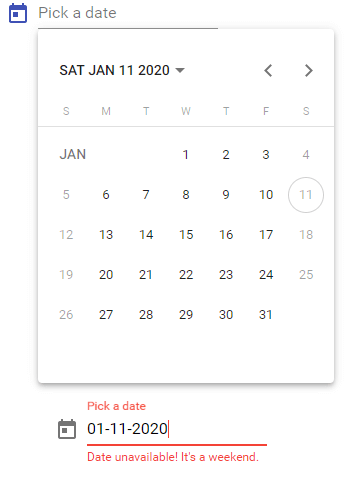The image depicts a pop-up calendar interface designed for selecting a date. At the top, there is a blue calendar icon accompanied by the text "Pick a Date." Immediately below this, a distinctive white box displays "Saturday, January 11th, 2020," with a downward-pointing arrow, indicating the option to change the date. 

Adjacent to this date box, left and right arrows allow navigation to the previous month, December, and the following month, February.

The calendar layout starts with Sunday and uses the abbreviations SMTWTFS for the days of the week: Sunday, Monday, Tuesday, Wednesday, Thursday, Friday, and Saturday. The focus is on January, with the 11th circled. Significantly, dates falling on weekends (Saturdays and Sundays) are grayscaled, denoting unavailability.

The bottom of the calendar features the text "Pick a Date" in red, and a grayed-out calendar icon emphasizes that January 11, 2020, is not selectable because it is a weekend. The annotation “Date Unavailable – it's a weekend” in red underlines that only weekdays are available for selection. This interface seems tailored for an establishment such as a dental office, which operates only from Monday to Friday, thereby rendering weekend dates unselectable.